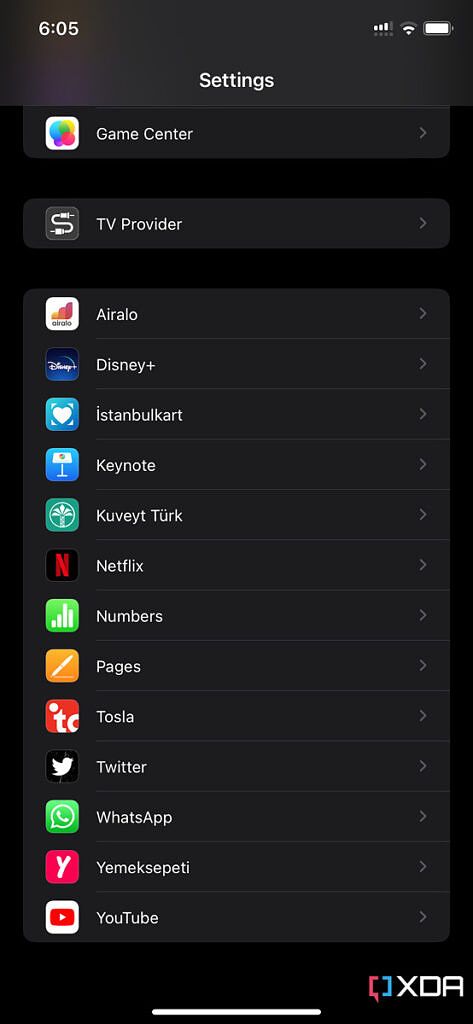Here's a concise and detailed caption for the image:

---

"Screenshot of the iPhone Settings app displayed in Dark Mode, showcasing a list of installed applications for customization. Visible apps include Game Center, TV Provider, Aerolo, Disney+, Istanbul Kart, Keynote, Kuvetserk, Netflix, Numbers, Pages, Tosla, Twitter, WhatsApp, Yemeksepeti, and YouTube. Each app entry features a right-arrow indicating access to individual settings. The top status bar displays the time (6:05), signal strength, Wi-Fi connection, and battery level. The bottom right corner features the text 'XDA' and a small icon, possibly indicating image source or tutorial guidance."